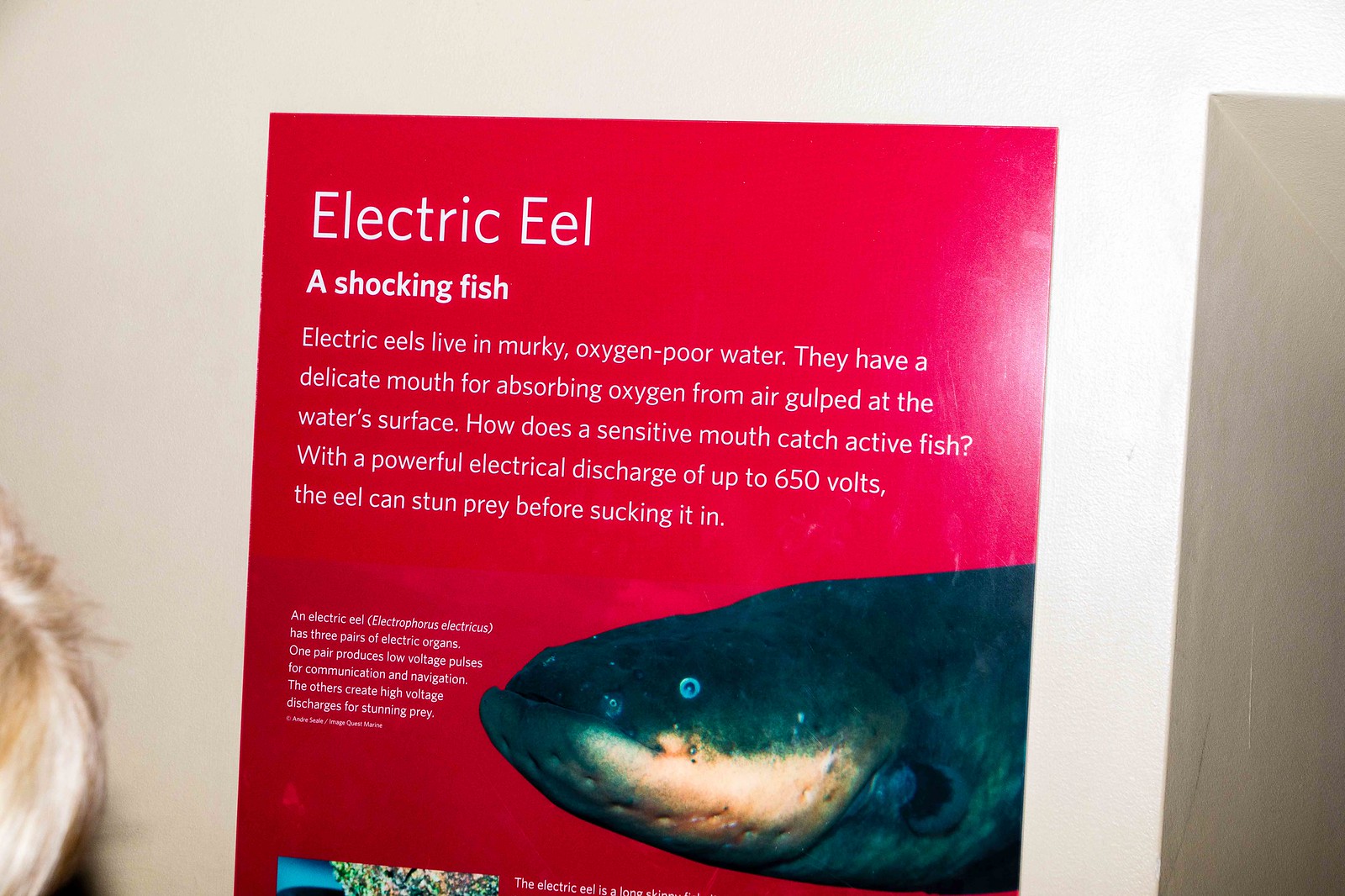The display is set against a neutral colored wall, probably white or off-white and appears to be something typically found beside an aquarium exhibit. At the center of the image is a bright red poster attached to the wall, detailing information about electric eels. Across the top of the poster, the text reads "Electric Eel" in a prominent white font, followed by the subheading "A Shocking Fish."

The main paragraph of the poster explains that electric eels reside in murky, oxygen-poor waters, utilizing their delicate mouths to absorb oxygen from the air gulped at the surface. It raises the question of how such a sensitive mouth catches active fish, answering that the eel employs a powerful electrical discharge of up to 650 volts to stun prey before sucking it in. Additionally, it clarifies that while the electric eel's shock is intense enough to stun a person, it is not lethal, akin to the experience of grabbing a live wire.

To the right of this informative text, there is an image of an electric eel, featuring greenish-teal skin, blue eyes, and a yellowish tint around its mouth. In the bottom right corner of the image, the eel's face and the first part of its body are prominently displayed. The bottom left of the image includes the top of a head with blonde hair, likely a viewer examining the display. Some additional text appears below the main description, but it is difficult to read.